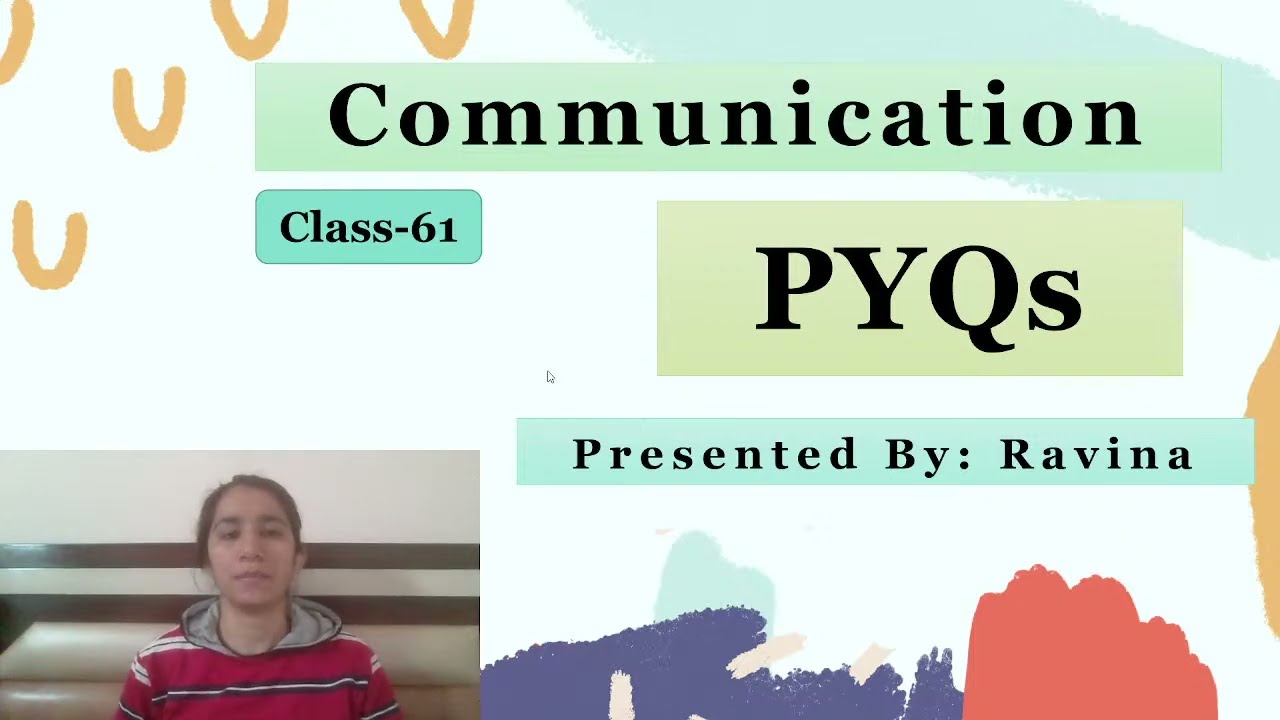The image resembles a PowerPoint slide designed with a mix of vibrant colors and informative text. The slide is rectangular and larger in width than height, reminiscent of a high-definition TV screen. Dominating the top center is the title "Communication," written in black text and enclosed within a lime-green rectangle. Just below the title, aligned to the left, is the text "Class 61" in black font within a slightly darker green, curved rectangle. Moving towards the center-right of the slide, there's a greenish-yellow block with large black letters spelling "PYQS," with the 'S' in lowercase. Beneath this, another green rectangle with black print reads "Presented by Ravina."

In the lower left corner of the slide, there is a photograph of Ravina, a young woman with light brown skin and straight dark brown hair pulled back in a ponytail with a side part. She is casually dressed in a red hoodie with white and black stripes, and the inside of the hoodie is gray. She is seated against a white wall with horizontal brown stripes, suggesting an indoor setting that could be a cozy area like a restaurant booth.

The slide's background is mostly light blue, adorned with several color splotches. The upper left corner features approximately five gold hues, while the top right corner has a streak of green paint. The lower right corner is decorated with splotches of purple, red, and green paint. Additionally, there's an off-centered gold swatch towards the far right of the slide. These artistic elements contribute to a visually engaging presentation design.